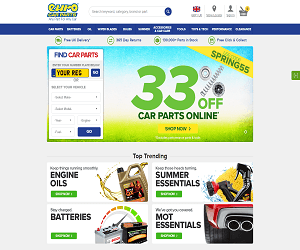The image appears to be a low-resolution screenshot of an e-commerce website focused on selling car parts. In the upper left corner, there's a logo, which might also be a stylized version of the business name, though it's unclear due to the resolution. Underneath the logo, there's a search box with a magnifying glass icon encased in a blue circle, although the placeholder text inside the search box is hard to read. Adjacent to this search box, there are multiple icons, some labeled with text.

A blue horizontal line separates the top section from the rest of the website. Below this line, there are several clickable links or perhaps descriptions of the service benefits, although the low resolution makes the text illegible.

The hero section of the website prominently features the call to action, "Find Car Parts," alongside input fields likely designed to help users search for specific items. This section includes a background image depicting a spring theme with green grass, a white horizon, and a blue sky. There’s a "33% off" banner for car parts, accompanied by a "Shop Now" button. In the upper right corner of the hero image, there’s a coupon code "SPRING55" displayed.

Towards the bottom of the page, there is a "Top Trending" section featuring four cards: Engine Oils, Summer Essentials, Batteries, and Mod Essentials. Each card likely represents a category of products available for purchase on the website.